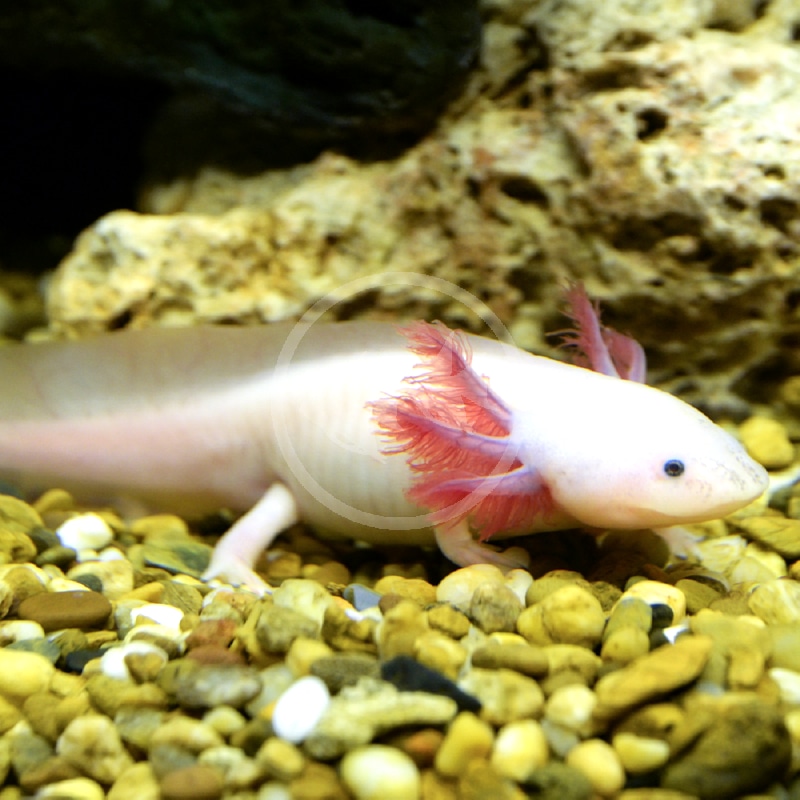The image depicts a slightly blurry, large square picture of an amphibian, likely an axolotl, captured from a side view. Central to the picture is the creature with an elongated body, a short snout, and a conspicuous small black eye located in the right middle area of the frame. The amphibian's head is predominantly beige, transitioning to a tanner shade towards its back, while the legs – of which there are four, two on either side – and underside remain beige.

Noticeably, the creature's distinctive gills, which resemble three feathery extensions on either side, are adorned with reddish-orange tendrils stemming from thicker purplish bases. This gives the appearance of an otherworldly aquatic organism.

The amphibian rests on a bed of small, pebbled stones that are primarily brown with sporadic white stones, hinting at a gold tint under certain lights. The photograph also showcases a porous rock formation in the background, occupying much of the upper middle and right side with its medium to light brown hues. The upper left corner of the image is defined by a solid black area, perhaps indicating the edge or background of an aquarium tank, which holds clear water. This detailed scene gives a glimpse into the intriguing life of this amphibious creature.